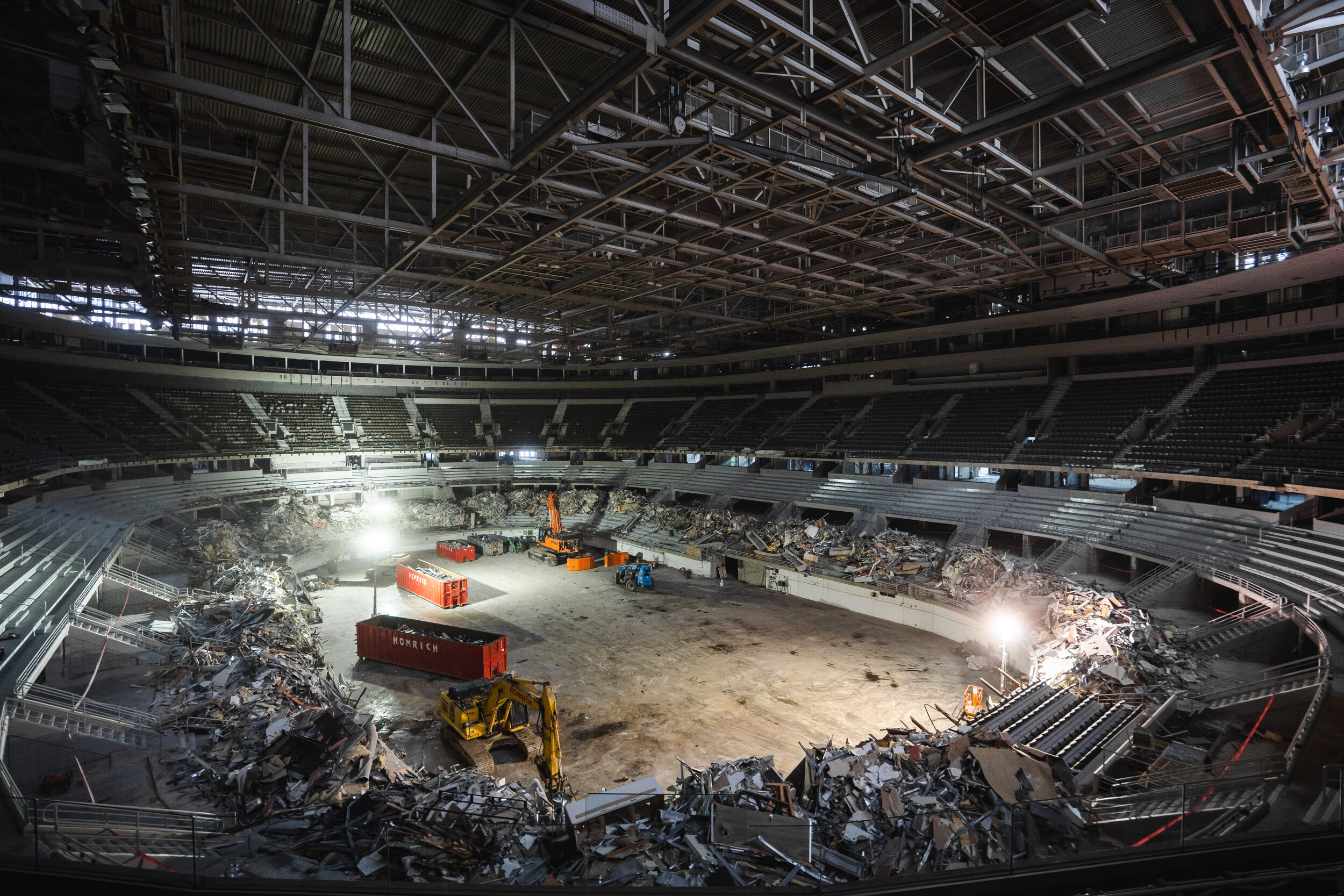The photograph captures the interior of a large indoor stadium undergoing significant demolition or possibly reconstruction. Viewed from a high vantage point, perhaps from the upper tier of seating, the image reveals a dark and cavernous space, illuminated sparsely by construction lights. Dominating the scene are rows of silver and gray bleacher-style seating that rises towards a grid-like network of steel beams supporting the roof.

On the floor of the stadium, a variety of construction equipment is scattered, including yellow caterpillar digger trucks and vibrant red and orange dumpsters. The central area, which might once have hosted a playing field or concert stage, is now filled with churned-up dirt and piles of debris. The first layer of seating appears heavily demolished, with concrete and metal rubble encircling the construction vehicles.

No workers are visible in the photograph, but the in-progress state of the project is evident from the torn seats, tilted bleachers, and construction materials. The color palette of the image is predominantly grayscale, with splashes of brighter hues from the machinery adding a stark contrast. The image overall suggests a transition phase for the stadium, either from active use to demolition or possibly towards a new structural purpose.